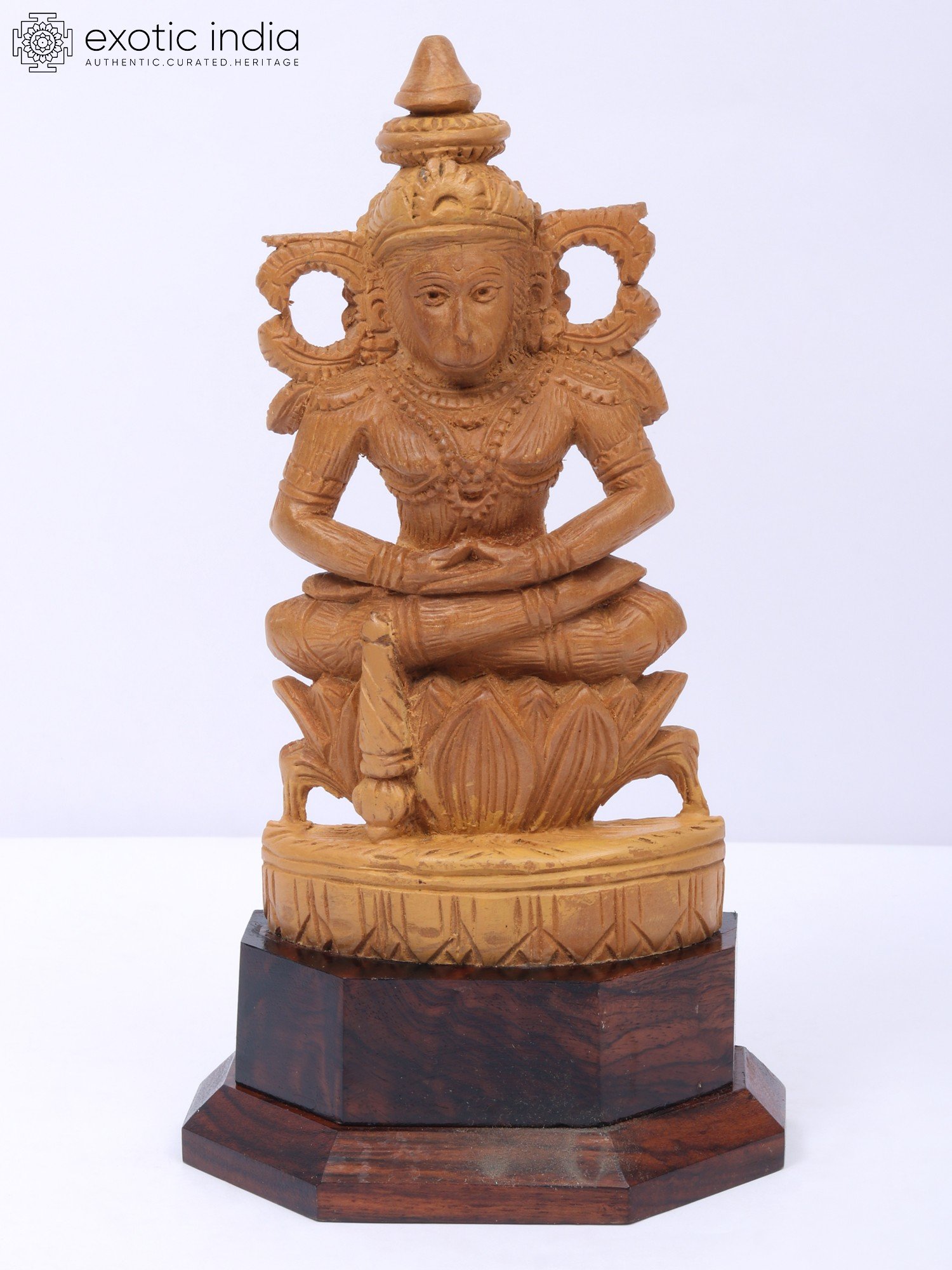The image depicts a small wooden statue, carved with impressive detail and polished to a fine finish, standing on a dark, reflective wooden base. The base supports another platform which the statue sits on. The statue features a person in a meditative position, seated with legs crossed and hands resting in their lap, with the left palm touching the bottom of the right hand and thumbs connected. The figure dons a beige v-neck garment adorned with bead-like details. Their head is crowned with a helmet that has two large circular elements on either side and comes to a point at the top. Behind the statue, on a white to cream-colored background, there's a black print that reads "Exotic India, Authentic Curated Heritage," accompanied by a small square logo with protruding marks and a circular pattern in the center.